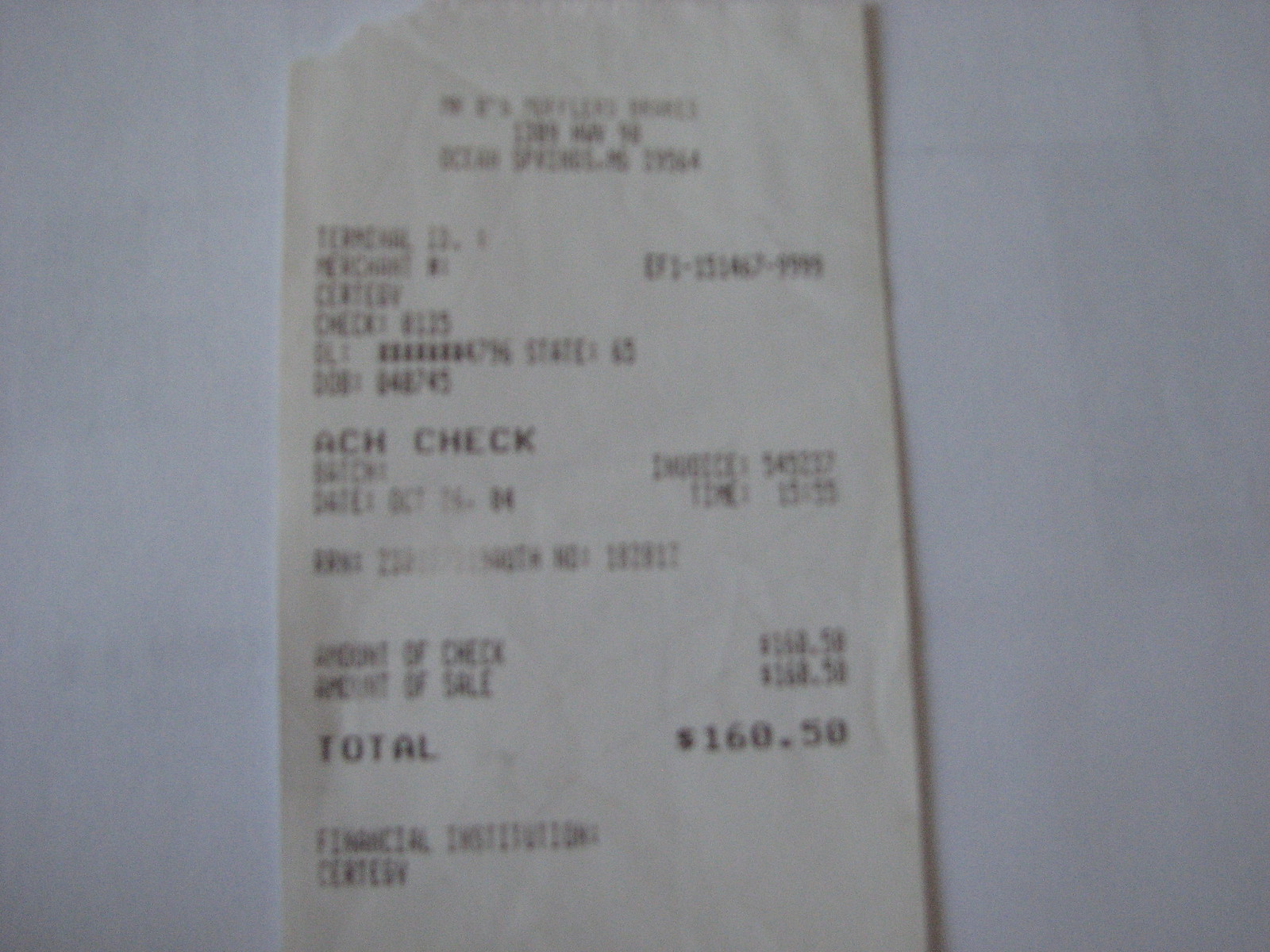This photograph depicts an off-white receipt, with black text, lying on a gray background. The text on the receipt is somewhat hard to discern, especially towards the top, where the specific name of the shop and address are nearly illegible. However, you can make out "Merchant ID" and "Terminal ID," followed by a partially obscured string of numbers that includes "EF1" and ends in "9999." The receipt mentions "Certigy Check 0123" and prominently features "ACH Check Invoice 141287" in bold print. Further down, it specifies a date stamp of October 14th, '04, and lists the fields "amount of check" and "amount of sale," with the total amount tallied to $160.50. Towards the bottom left, it references the financial institution Certigy, though some words remain indistinguishable due to the blurred quality of the image.